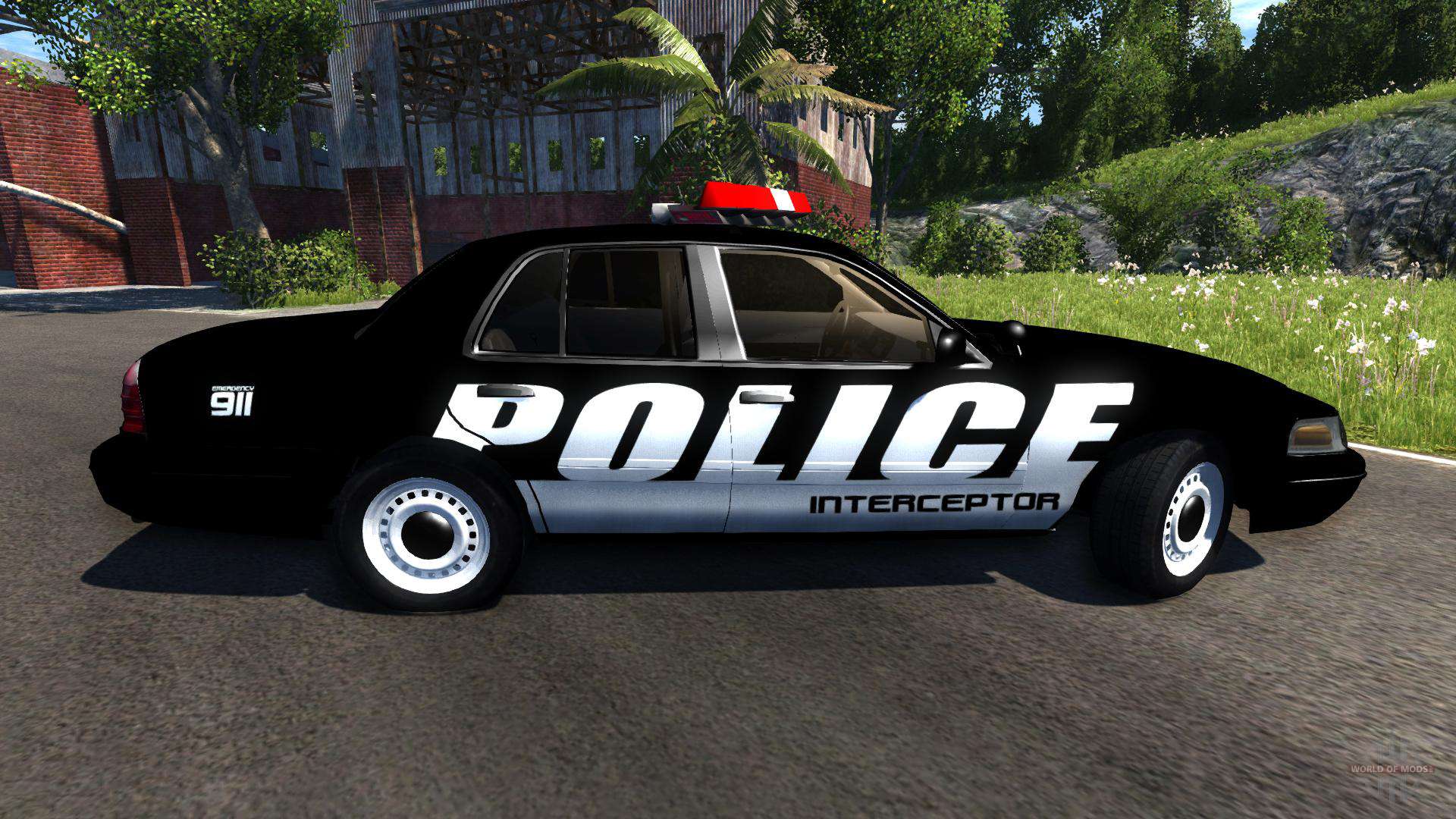The image is a detailed digital rendering reminiscent of a video game environment, featuring a prominent black and white police interceptor with red and white lights centered in the scene. The side profile of the vehicle displays distinctive text: "POLICE INTERSECTOR" in white, italicized, and all-caps font across the doors, with "911" marked on the rear left panel. The car is positioned on a gray paved road, with its front tire turned to the left. Surrounding the police car is a vivid environment with various elements: 

- **Top Right:** Rocky terrain leading up a hill, interspersed with grass and trees, including a tall palm tree and other tropical foliage.
- **Bottom Left:** The gray road extending from beneath the car.
- **Center Above Car:** A large, dilapidated building with glass and brick walls, supported by concrete and metal structures, indicative of a warehouse or industrial style.
- **Background:** A mixture of green grass, white wildflowers, and additional trees, enhancing the summertime, warm climate ambiance. The sky is brightly rendered, adding a sunny feel to the scene.

With intricate attention to detail, from the textures of the building to the layout of natural elements, this image captures an immersive, explorable 3D-rendered world.